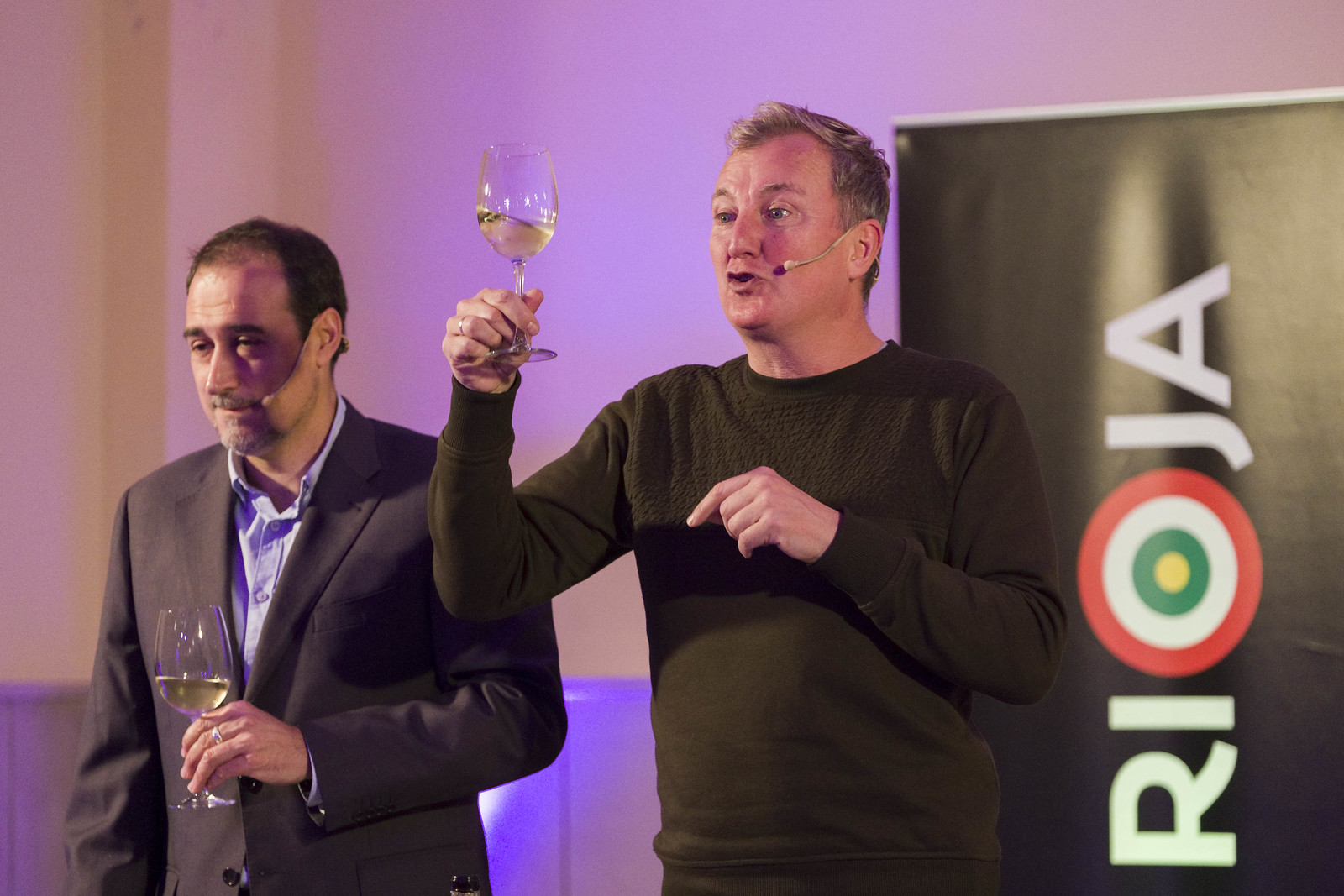In a well-lit room, two men with headset microphones are standing on a stage in front of a white background featuring a Rioja sign. The sign has green letters for 'Ri', a target design for the 'O', and white letters for 'ja'. The man on the right has blonde hair and is dressed entirely in black, including a black sweater. He holds a glass of champagne in his left hand, showcasing a ring on his wedding finger, while his right hand is raised to shoulder height as he appears to be speaking. Beside him, to the left, is a man with dark hair wearing a brown suit jacket over a light blue collared shirt. His suit jacket is open, and he holds a wine glass at waist-level in his left hand, also displaying a ring. Both men are standing calmly, engaged in what appears to be a presentation or discussion.